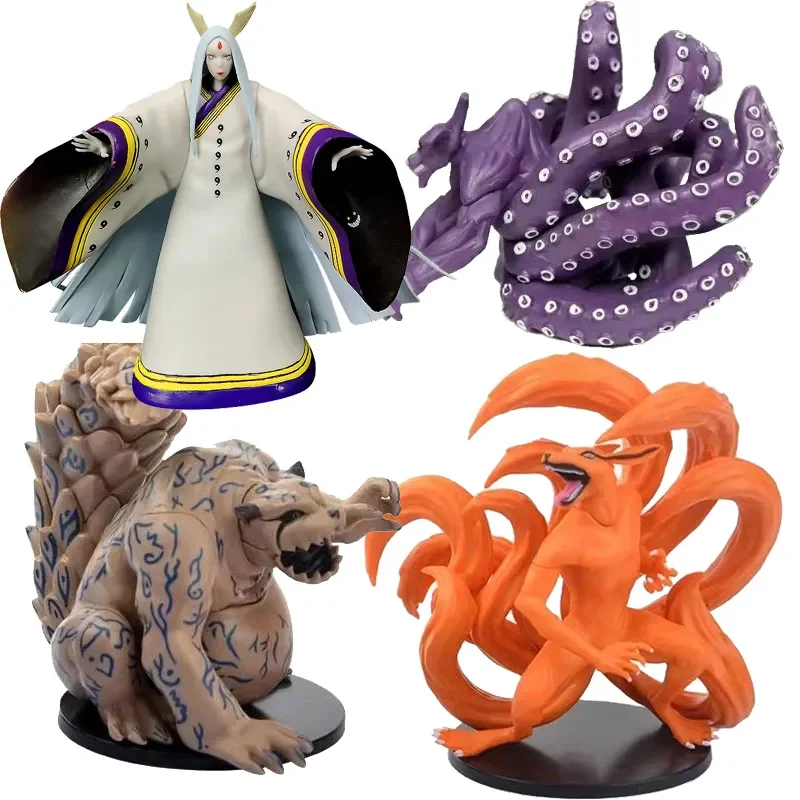The image displays a captivating collection of four distinct action figures, each occupying one corner of the frame. In the top-left corner is an elegant, enigmatic female figure adorned with long, dagger-like beige horns and a light blue hair cascading down. She is garbed in a flowing white robe detailed with purple and yellow trim, and a small red dot marks her forehead. To her right, on the top-right side, a muscular imp-like creature with five visible white tentacles coils around its purple, octopus-like body, reminiscent of a hybrid gargoyle. The bottom-left corner features a large, squirrel-like creature with a substantial belly and a significantly large tail, embellished with light dark blue markings. In the bottom-right corner stands a many-tailed red fox, its ears large and expressive. It has a ferocious expression with an open mouth and its tongue hanging out, projecting an aura of readiness and vitality. This compelling display of figures could serve as collectible statues or artistic toys, each brimming with intricate details and unique characteristics.